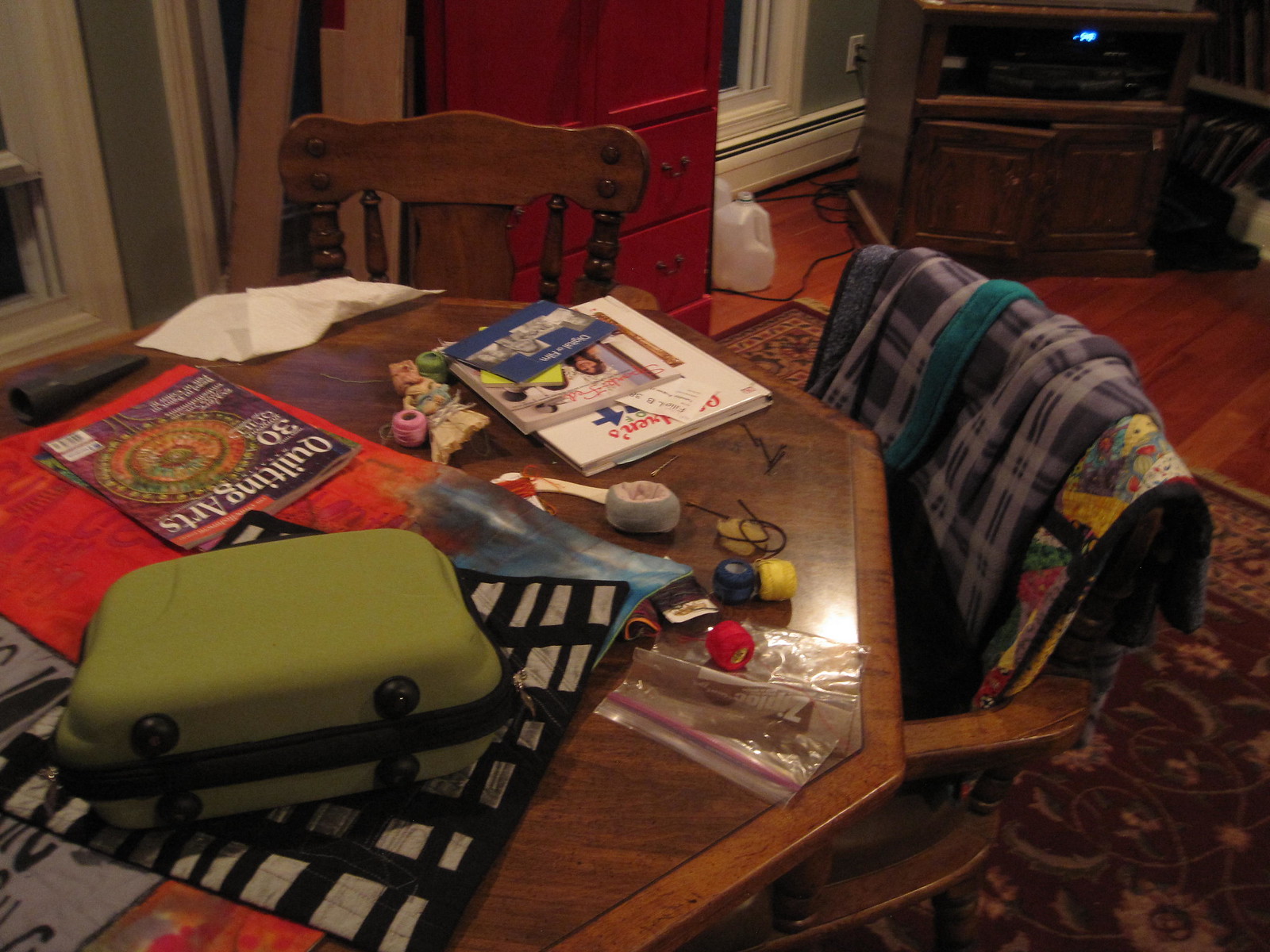In the background of the image, there is a large, dark wooden cabinet with drawers featuring metal handles. A plastic jar can be seen at the bottom of the cabinet, while the top right section reveals a slightly open door. In the foreground, there is a table displaying an open magazine titled "Quilting Arts," featuring a colorful circle design and a prominent pink jar in the center. Scattered papers and a green container are also visible on the table. Below these items, part of a quilt and several spools of thread in blue, yellow, red, and pink can be seen. Additionally, a bracelet, a small doll, and a stack of books are arranged nearby. In the background, a wooden chair is positioned against the wall, while a chair on the right side of the image is draped with a blue blanket adorned with white squares and black stripes, and a vibrant, colorful blanket in shades of yellow, green, black, and red. A large rug extends across the floor, completing the scene.